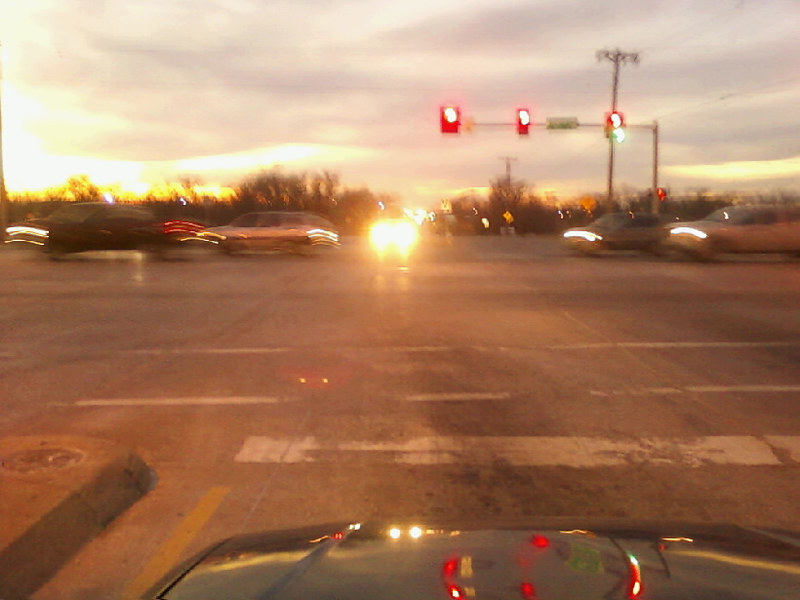The image depicts a busy road scene during the late evening as the sun is setting, casting a yellow glow along the tops of the trees beneath a sky covered in clouds. The photo, seemingly taken from the front seat of a car through its windshield, shows the hood of a light green vehicle with the reflection of red stoplights clearly visible. In the distance, traffic lights are mounted on a pole, with all lights currently red and spaced about a foot or two apart. The intersection ahead features bright yellow headlights of another car facing towards the camera, creating a striking contrast with the overcast sky. Several cars are captured moving horizontally across the frame from right to left, their headlights blurred but discernible. White and somewhat faded parking lines are visible on the pavement, and at the horizon, a blend of trees and road signs, including a few yellow ones, can be seen alongside the traffic lights. Despite the blurriness, the photograph vividly conveys the busy and atmospheric nature of this evening scene.